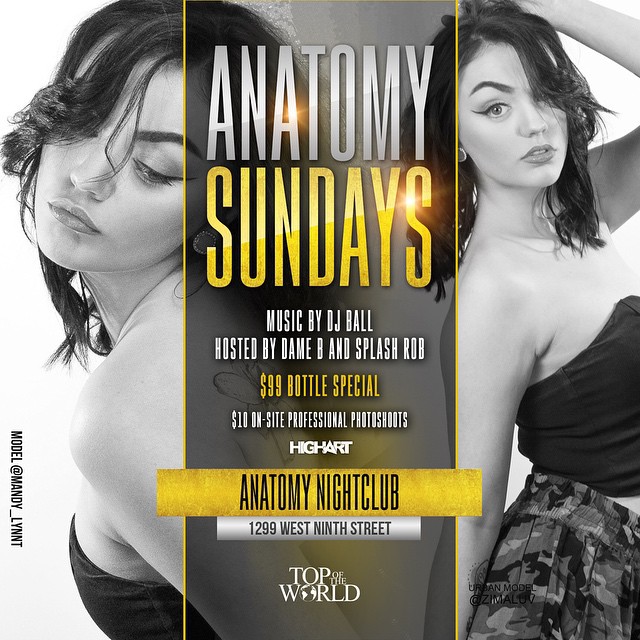This square advertisement poster features two black and white photographs of the same brunette woman with curly hair. On the left side, she is posed from the torso up, turned to her left with her head forward and eyes downcast, wearing a black tube top. On the right side, she faces her body rightward with her head looking straight ahead, striking a seductive pose. Between and in front of these images is a gray column with gold borders, prominently displaying the event title "ANATOMY SUNDAYS," where "Anatomy" is in silver and "Sundays" in gold. 

Beneath these details, the poster advertises a $99 bottle special, $10 on-site professional photo shoots, and a high art experience. The event is hosted by DJ Ball, Dane B, and Splash R.O.B., taking place at Anatomy Nightclub located at 1299 West 9th Street, with a special mention of "Top of the World." The poster also features the Instagram handle of the model, suggesting attendees might meet someone like her at the event.